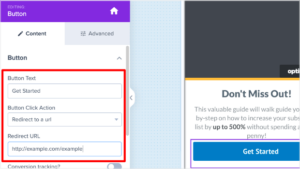The image features two distinct screenshots. The first screenshot displays a red box with a purple banner at the top. The red box appears to be highlighting an area of the screen, but the text within it is too small to read. In the middle of this screenshot, there is a baby blue banner with the text "Don't miss out" on the right side. Next to this text is a blue button that says "Get Started." However, the details and content of the highlighted sections and the button text are not legible due to the small size of the images.